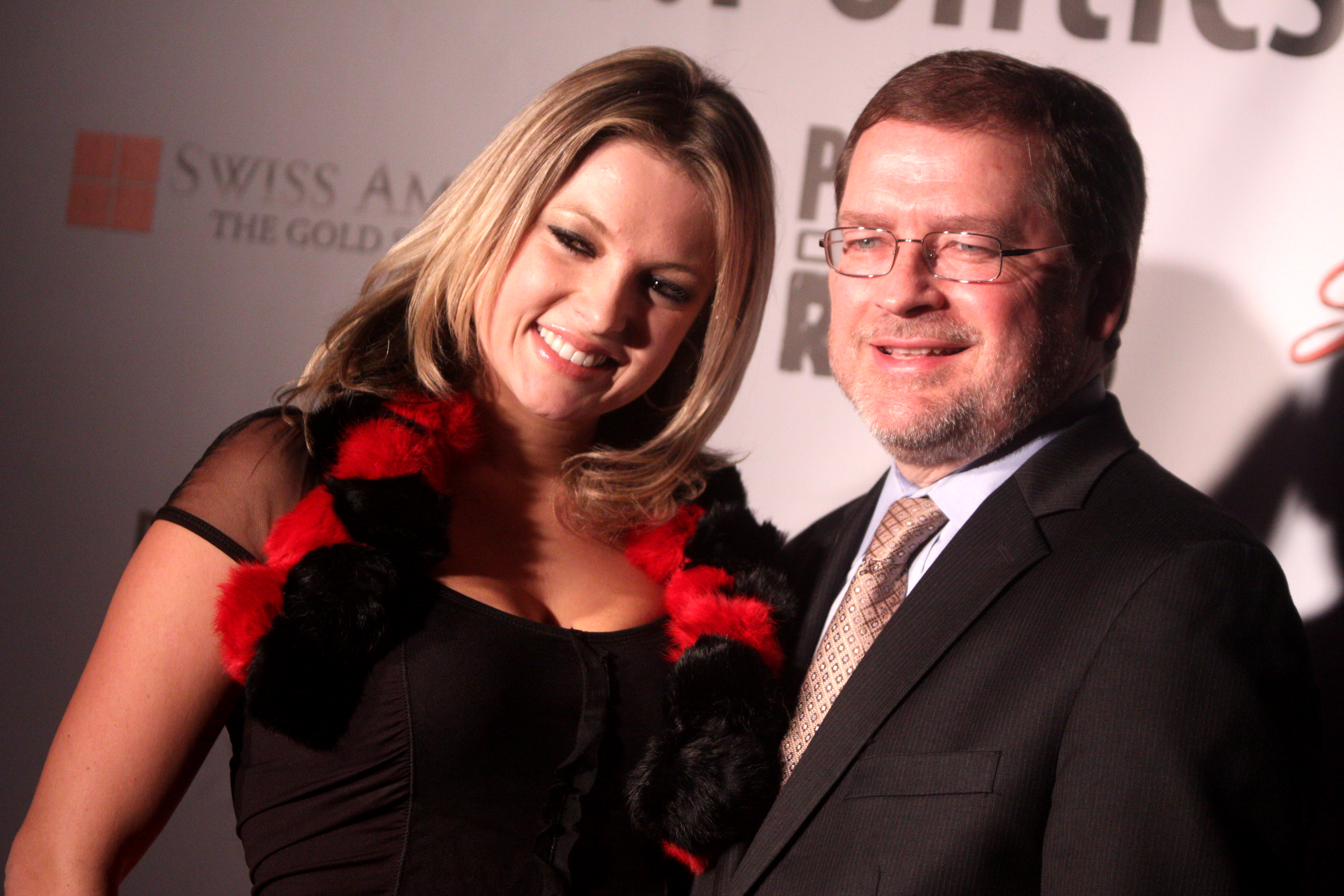In this red carpet event photograph, two individuals, a woman and a man, are captured in front of a white banner adorned with gold lettering and multiple logos. The visible text on the banner includes "Swiss AM" and partially obscured words, with a coral-colored box to the left. The woman, positioned on the left side of the image, has shoulder-length blonde hair and is smiling while looking slightly off to the side. She is dressed in a black, low-cut dress featuring mesh on the shoulders and accessorized with a black and red bow around her neck. Her right arm is down and slightly out to her side, and the image cuts off above her waist. To her right stands the man, who has short brown hair and wears gold-framed glasses. He is also smiling, facing the same direction as the woman. He is dressed in a dark suit jacket, a white shirt, and a gold tie with diamond patterns. His hand appears to be wrapped around the woman's back, suggesting a close or affectionate stance. Behind the man, additional parts of the banner and logo are partially obscured, blending into the scene.